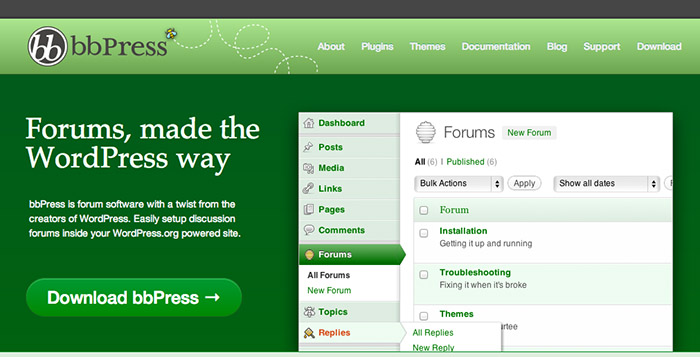Screenshot of a Website Highlighting bbPress Features and Navigation

The screenshot showcases the homepage of the bbPress website. In the upper left corner, the iconic bbPress logo is prominently displayed next to a whimsical graphic of a bee in flight. The primary navigation bar includes menu items such as "About," "Plugins," "Themes," "Documentation," "Blog," "Support," and "Download."

On the left sidebar, a bold headline reads, "Forums made the WordPress way." Below this, a brief introduction to bbPress describes it as a unique forum software developed by the creators of WordPress. The software is designed to seamlessly integrate discussion forums into any WordPress.org-powered site. 

A prominent green button labeled "Download bbPress" invites users to start the installation process.

To the right, the user interface menu includes options like "Dashboard," "Posts," "Media," "Links," "Pages," "Comments," "Forums," "All Forums," "New Forum," "Topic," and "Replies."

Further down, detailed forum management options are listed, such as "Forums," "New Forum," "All," "Published," and tools like "Bulk Actions" and "Apply." Specific sections are dedicated to forum tasks: "Installation," "Getting it up and running," "Troubleshooting and fixing it when it's broke," "Themes," "All Replies," and "New Reply."

The layout and detailed options underscore the comprehensive functionality bbPress offers for managing discussion forums within WordPress.